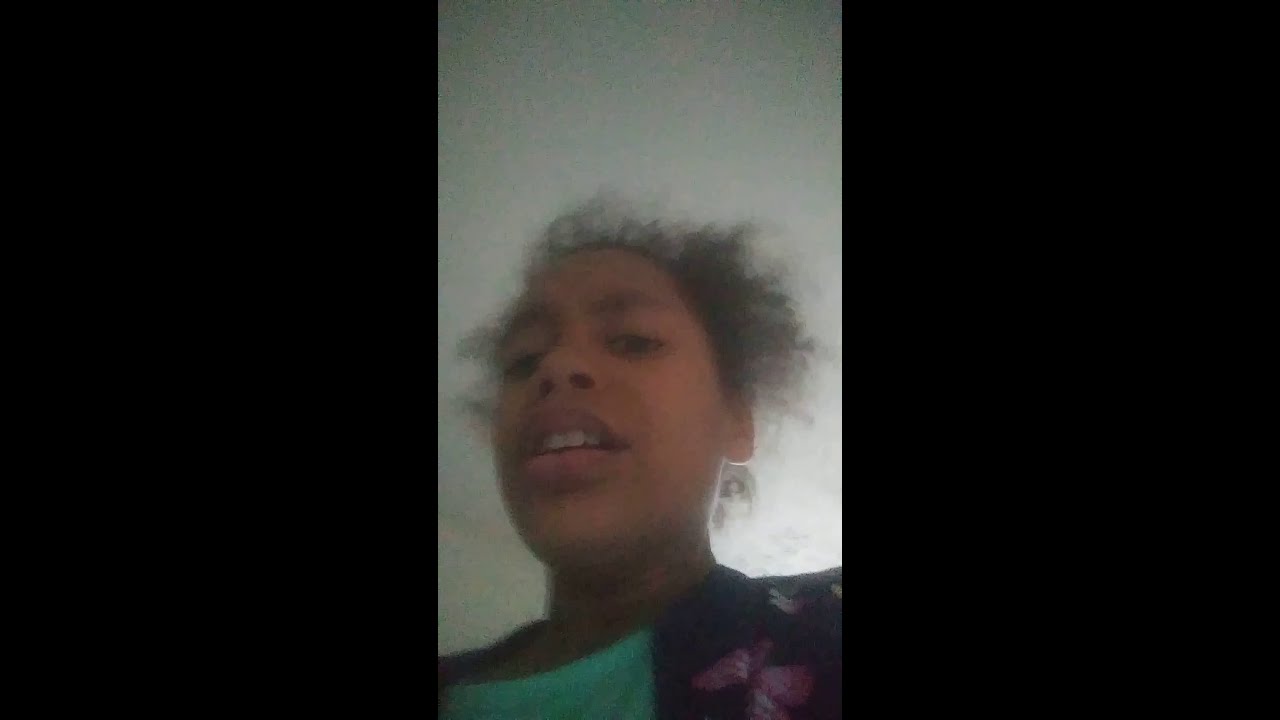The image depicts a black woman in a dimly lit room, captured in a vertical photo framed by solid black panels on either side, suggesting a still from a video. Her frizzy, dark hair stands up slightly, and she's looking down at the camera with an expression that could be interpreted as surprised or stressed, evidenced by her slightly open mouth. She wears a mint green shirt that's partially visible under a dark purple over-shirt adorned with a pinkish-purple butterfly design. The background features grayish-white walls and a ceiling, contributing to the room's dim ambiance. A single dangly earring can be seen on one ear, catching some light from the background. The overall image is horizontally oriented, with the detailed vertical snapshot of the woman centered in the middle.